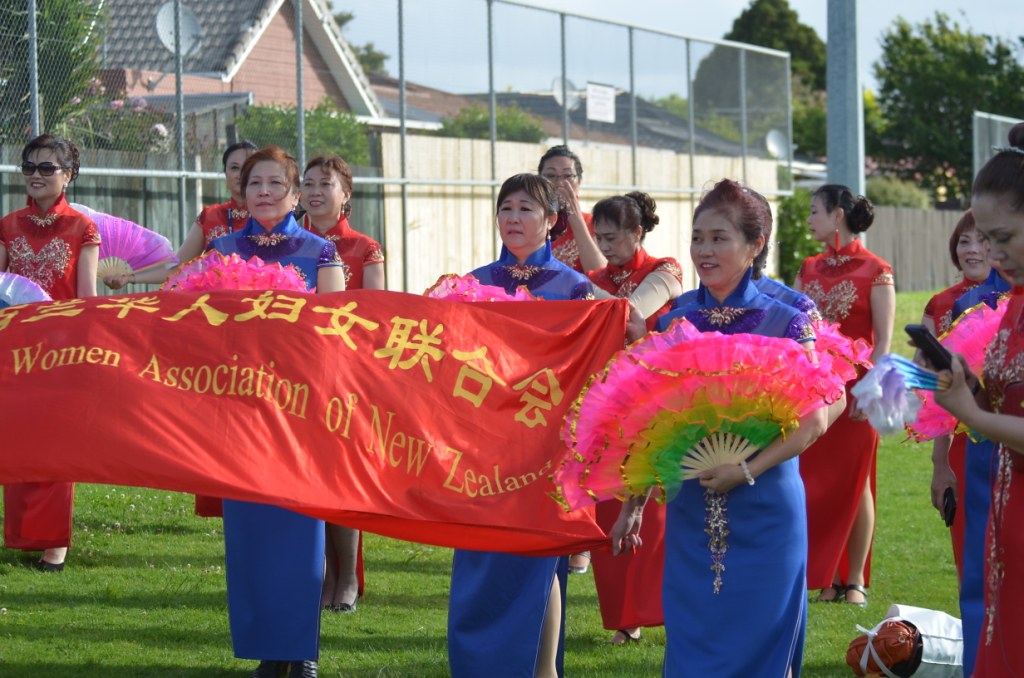In this vibrant photograph taken outdoors in a scenic park, a group of women stands proudly on a well-manicured field of green grass. The background reveals a residential area with houses, wooden fences, and a chain-link fence adorned with three satellite dishes, all under the canopy of lush trees.

The women are elegantly dressed in long robes, some in red and others in blue, all featuring intricate gold embroidery along the center, sleeves, and collars. They hold vivid, rainbow-colored fans in hues of pink, green, yellow, and purple, adding a burst of color to the scene. Prominently in the front, women in blue gowns hold up a silk banner. The banner is inscribed with Asian characters in gold at the top, and beneath, in English, it reads "Women Association of New Zealand." This picturesque moment captures the elegance and cultural richness of the gathering.